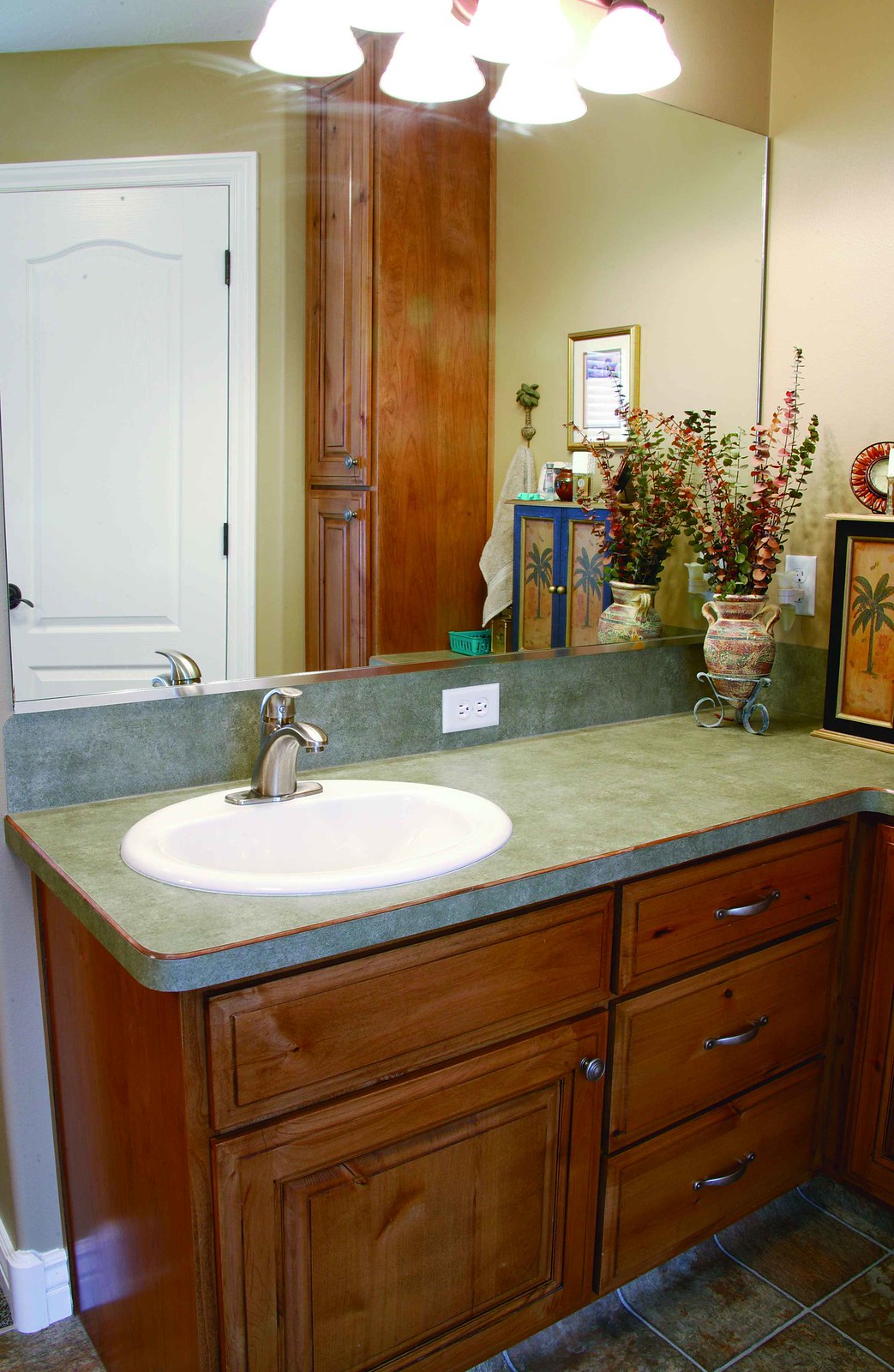This image depicts a meticulously detailed interior shot of a restroom. At the very top, there are four intensely bright lights that illuminate the space. Beneath these lights, a large mirror reflects the back of a substantial white wooden door, adorned with a dark handle and visible hinges at the top and middle.

To the right of the door, the reflection reveals two substantial cabinets, side-by-side. The left cabinet features two doors—one on the top, one on the bottom—each adorned with rectangular designs and handles. The cabinet itself is characterized by its rounded and curved walls.

To the right within the reflection, a painting hangs on the wall, showcasing a beach scene with a palm tree in a drawn illustration style. Below this artwork, decorations include a charming vase with a handle on each side, crafted from clay with specks of white or gray. The vase is filled with a vibrant arrangement of red and green flowers that look as if they might be aromatic.

Dominating the lower half of the image is a sleek grayish countertop, complete with a pristine white porcelain sink and a shiny silver faucet. Beneath the sink, there's a drawer and a substantial cabinet, along with three rectangular drawers on the left, each accented with a silver handle situated in the center. The entirety of the floor is covered in elegant black tiling, grounding the scene with a touch of sophistication.